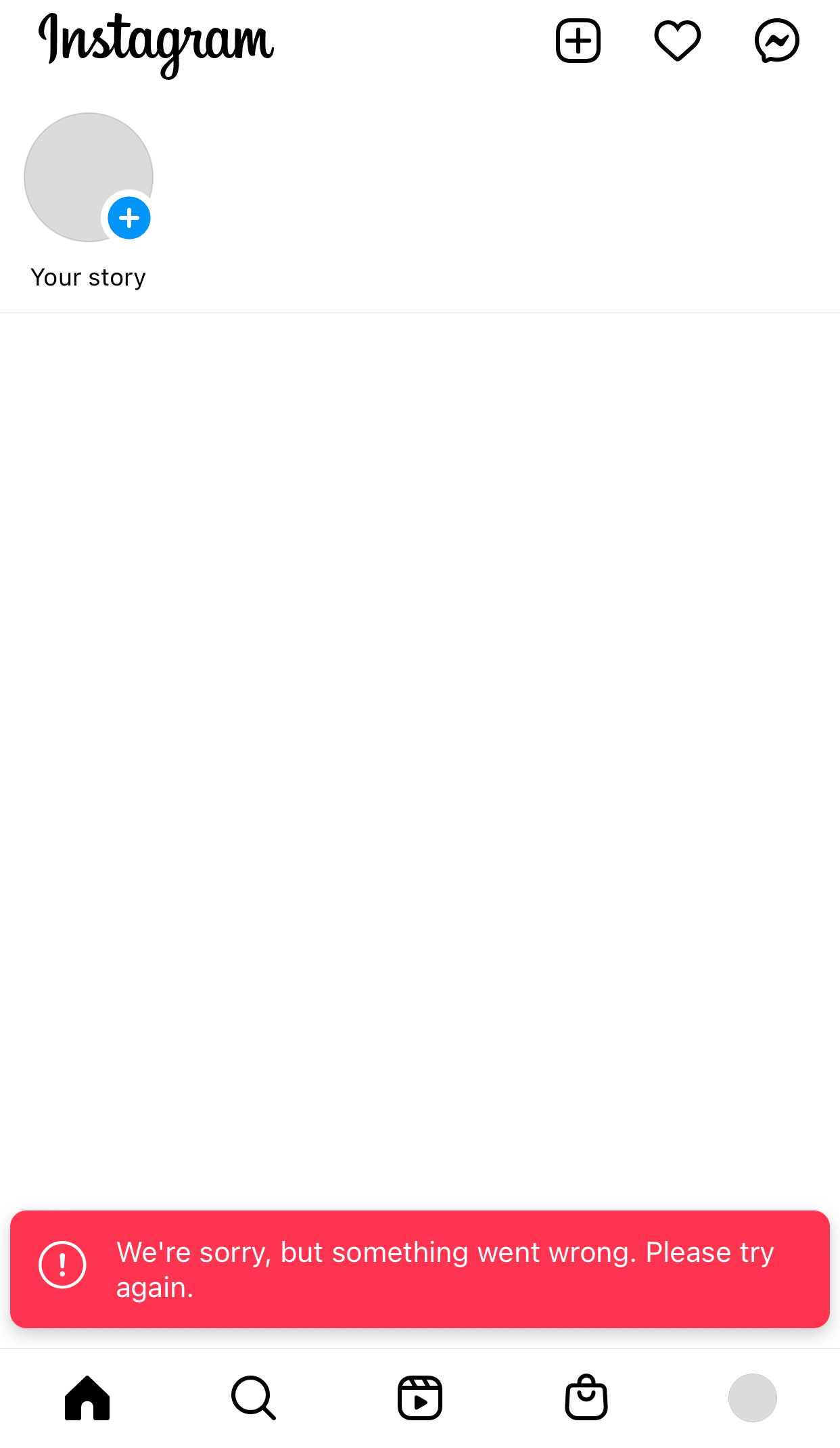This image features a user interface with a white background. At the top, there is an Instagram logo, followed by a series of icons: a black square with a plus sign, a heart, and a messenger symbol. To the right, there is a gray circle containing a blue circle with a white plus sign, likely indicating the "Add to Your Story" function. Below these, a red rectangle with a white circle and an exclamation mark displays an error message stating, "We're sorry, but something went wrong. Please try again." Towards the bottom of the image, additional navigation icons are visible: a house, a magnifying glass, a square with a triangle (possibly a camera or media icon), and a shopping bag, complemented by another gray circle.